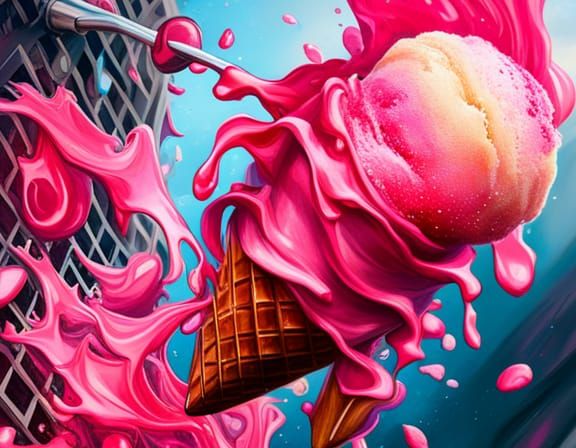The image is a detailed and vibrant colored drawing, almost with an animated feel, depicting an ice cream cone amidst a dynamic and somewhat chaotic scene. Dominating the right side, the cone begins at the bottom left of center, extending upward and to the right. The cone itself, while only partially visible, is a classic waffle cone characterized by crisscrossing squares and triangles. 

Above the cone, a mix of pink swirls, resembling either melty or soft-serve ice cream, cascades upward and to the left. This pink swirl theme continues throughout the image, adding a sense of motion as it flows through and around the cone, contributing to an impression that the ice cream is in the process of a dramatic meltdown.

At the top of the cone, in the upper right of the image, sits a scoop of ice cream with a gradient from pink at the bottom to white on top, and streaked with additional pink. This scoop adds to the visual interest as pink swirls extend from it both upwards and downwards, suggesting movement and splatter.

The background accentuates the scene with varying tones of blue and green, particularly evident in the bottom right corner. On the left side of the image, spilling beneath and around the cone, more pink swirly ice cream is visible, amplifying the sense of messiness.

Interestingly, the leftmost side and top left corner of the image feature a gray, grid-like structure with small squares and bars that resemble a metal grill or grate. This possibly tube-shaped grill extends across the canvas, creating a contrasting backdrop against which the ice cream cone appears to splatter.

The entire composition is presented in landscape orientation, blending 2D and elements that give it a slightly 3D appearance, encapsulating a scene of delicious chaos with its melting ice cream and vibrant splatters.